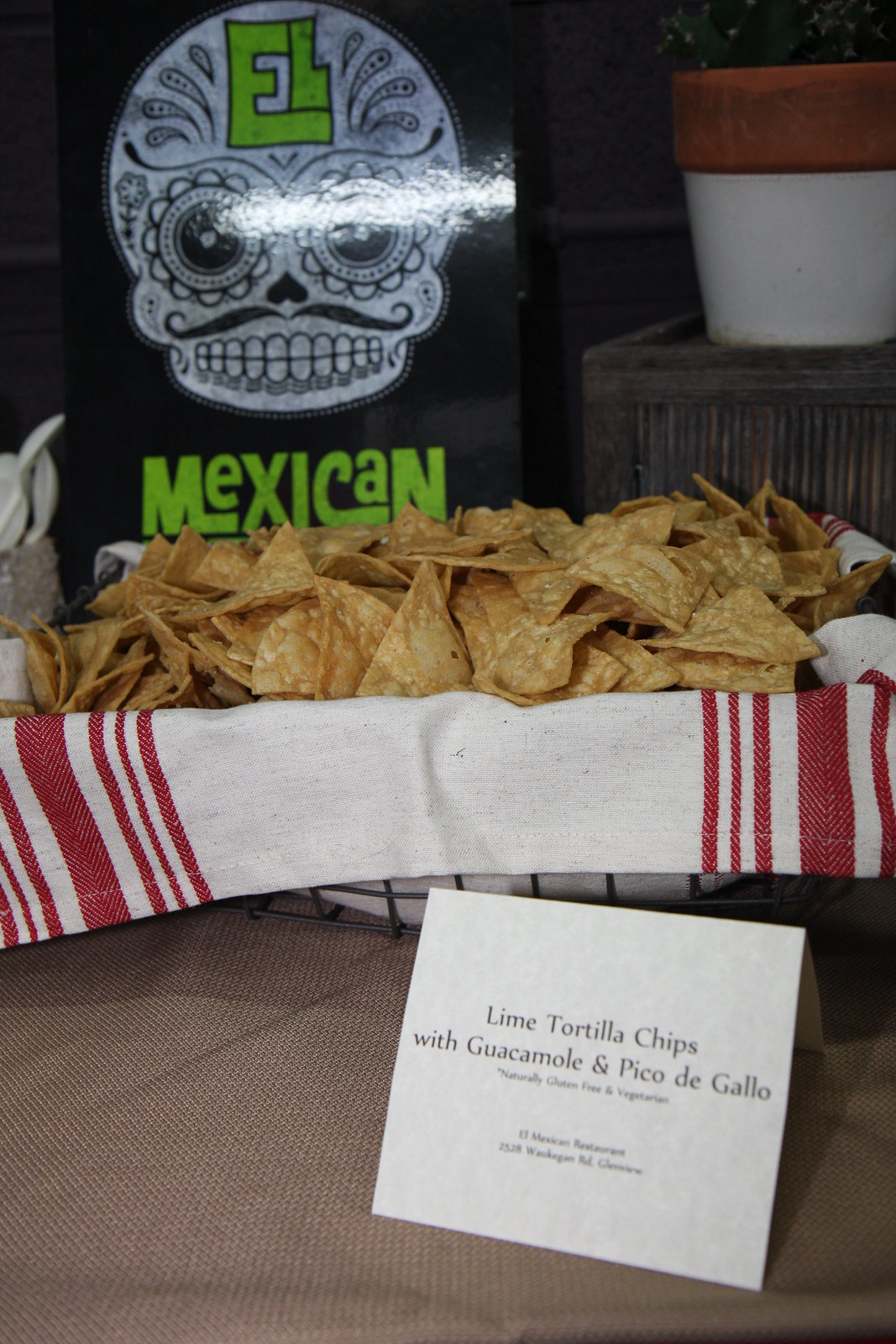The image features a basket of tortilla chips prominently placed in the center, lined with a white and red striped cloth. At the bottom right, a white postcard rests on a tan fabric, displaying the text "Lime Tortilla Chips with guacamole and pico de gallo." In the background, there is a striking black sign with a stylized skull adorned with large eyes and green lettering that reads "El" above the skull and "Mexican" below it. The upper right corner of the image shows a clay and white flower pot with some plants. The setting appears to be indoors at a festive gathering, with the vibrant colors and decor enhancing the lively atmosphere.